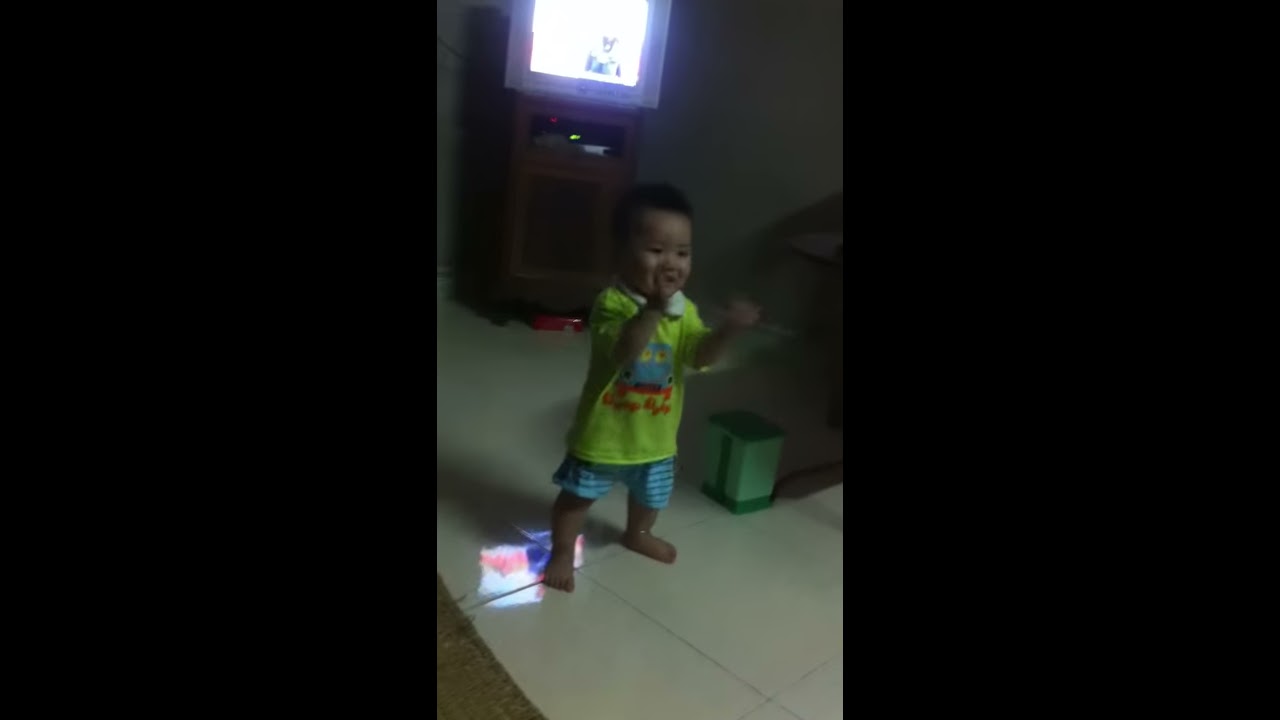In this dimly lit indoor photograph, a young Asian toddler, possibly one to two years old, stands barefoot in the middle of a living room. The child, whose dark, short hair suggests they might be a boy, wears a bright yellowish-green shirt adorned with an indiscernible design in red lettering and light blue, horizontally striped pants. A blend of white and red light casts a glow on the toddler’s leg and foot, which are reflected on the tiled floor beneath them. Behind the child, a television screen mounted on a TV stand illuminates the room, adding a sharp contrast to the otherwise dark setting. Beside the toddler, a green box-shaped object and a faintly visible chair contribute to the cluttered yet homely atmosphere. Black rectangles frame the photo on either side, focusing attention on the joyful child who appears to be smiling, likely engaging with a family member out of the frame. A red object is noticeable on the floor underneath the television, adding a pop of color to the scene.